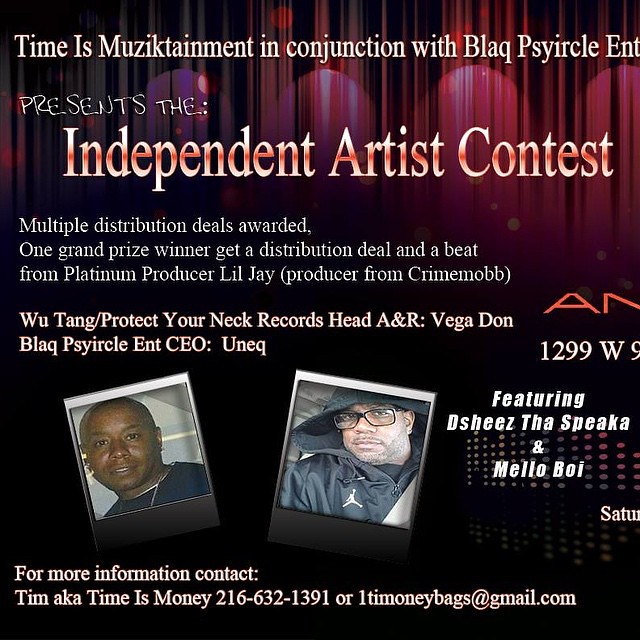The image is a promotional poster for an event titled "Independent Artist Contest," organized by "Time is Musictainment in conjunction with Black Circle Entertainment." The background features a dark, mainly black hue with red or purple curtains at the top, resembling a stage presentation. Prominently displayed in white and orange letters, the poster announces multiple distribution deals to be awarded, with a grand prize including a distribution deal and a beat from platinum producer Lil J of Crime Mob. Additional credits highlight Wu-Tang's Protect Ya Neck Records' Head of A&R, Vegadon, and Black Circle Enterprises' CEO, Eunik.

The poster also showcases two small, Polaroid-like photos of hip-hop artists. One artist, identified as Desheez The Speaker, is wearing a black shirt without a collar, while the other, named Mellow Boy, is dressed in a black jacket with a white insignia on the front. For further details, viewers are directed to contact Tim, aka TimeIsMoney, at 216-632-1391 or via email at onetimmoneybags@gmail.com.